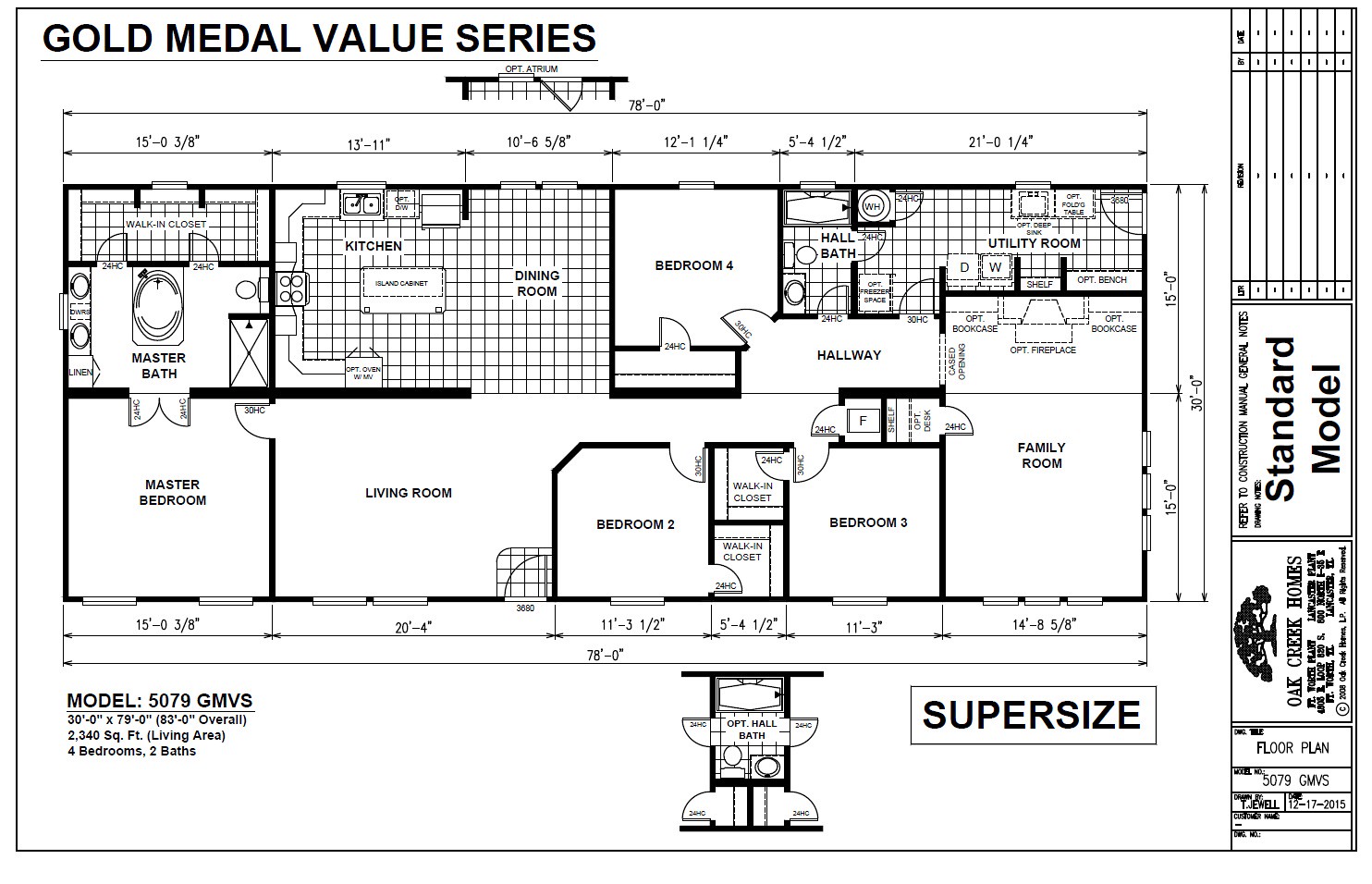The diagram depicts a detailed floor plan of a one-story home, labeled as Model 5079 GMVS, drawn in black ink on white paper. With the Gold Medal Value Series trademark in the upper left corner, this layout showcases a practical and elegant design. The total living area spans 2,340 square feet, featuring four bedrooms and two bathrooms. 

Starting from the lower right, the family room provides a welcoming space for gatherings. Moving left, Bedroom 3 is conveniently located adjacent to a shared bathroom. Next to this, Bedroom 2 boasts its own private bathroom. The living room, situated further to the left, serves as the central hub of the home, with the master bedroom nestled just to its left. The master bedroom has direct access to the master bath, positioned in the upper left corner of the diagram.

The kitchen and dining area are situated to the right of the master bath, offering a functional and central place for meals and socializing. Adjacent to the dining area is Bedroom 4, complete with its own bathroom. The utility room, designed for laundry needs, is located to the far right, next to an office space equipped with a fireplace for a cozy work environment. A connecting hallway runs through the home, ensuring easy access to each room.

Additionally, the diagram includes a note about an optional hall bath, positioned below the main floor plan, indicating a flexible option to add an extra bathroom for enhanced convenience.